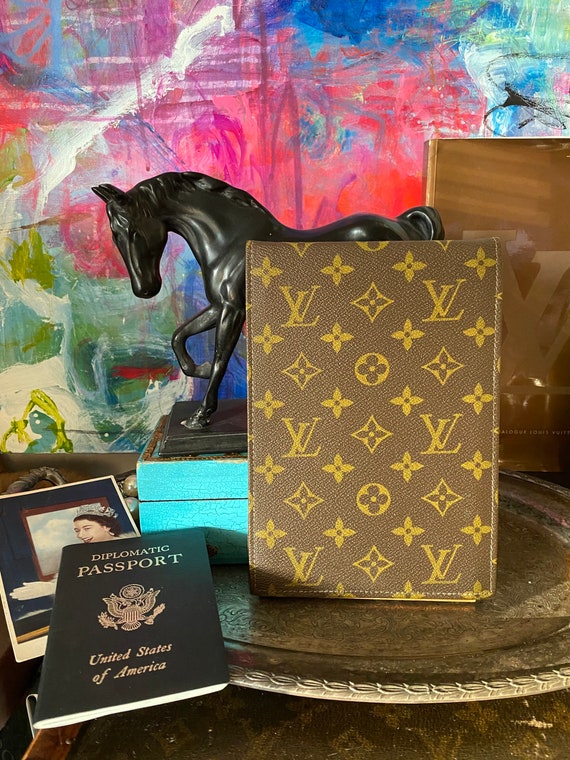The photograph shows a collection of various objects arranged on a brown surface, possibly a table or desk, with a wooden edge visible at the bottom left. Central to the frame is a metal dish, oval-shaped, upon which most items are placed. On this dish, prominently positioned right of center, is a standing Louis Vuitton leather-bound book, adorned with orange floral patterns and the LV logo.

To the left of this notebook and still on the platter, there is a brown and blue wooden box. Perched atop this box is a black metal statue of a horse, facing left with one front hoof raised. 

To the far left edge of the platter lies a black diplomatic passport bearing the gold-embossed text "Diplomatic Passport, United States of America." Partially tucked beneath this passport is an image of a young Queen Elizabeth, wearing a crown and white gloves, set against a backdrop suggestive of a window.

Behind these items, occupying the background, is a colorful abstract painting. The artwork features a mishmash of colors, including reds, blues, greens, pinks, purples, whites, and yellows, with a possible depiction of a person with yellow hair located at the left-center of the entire image.